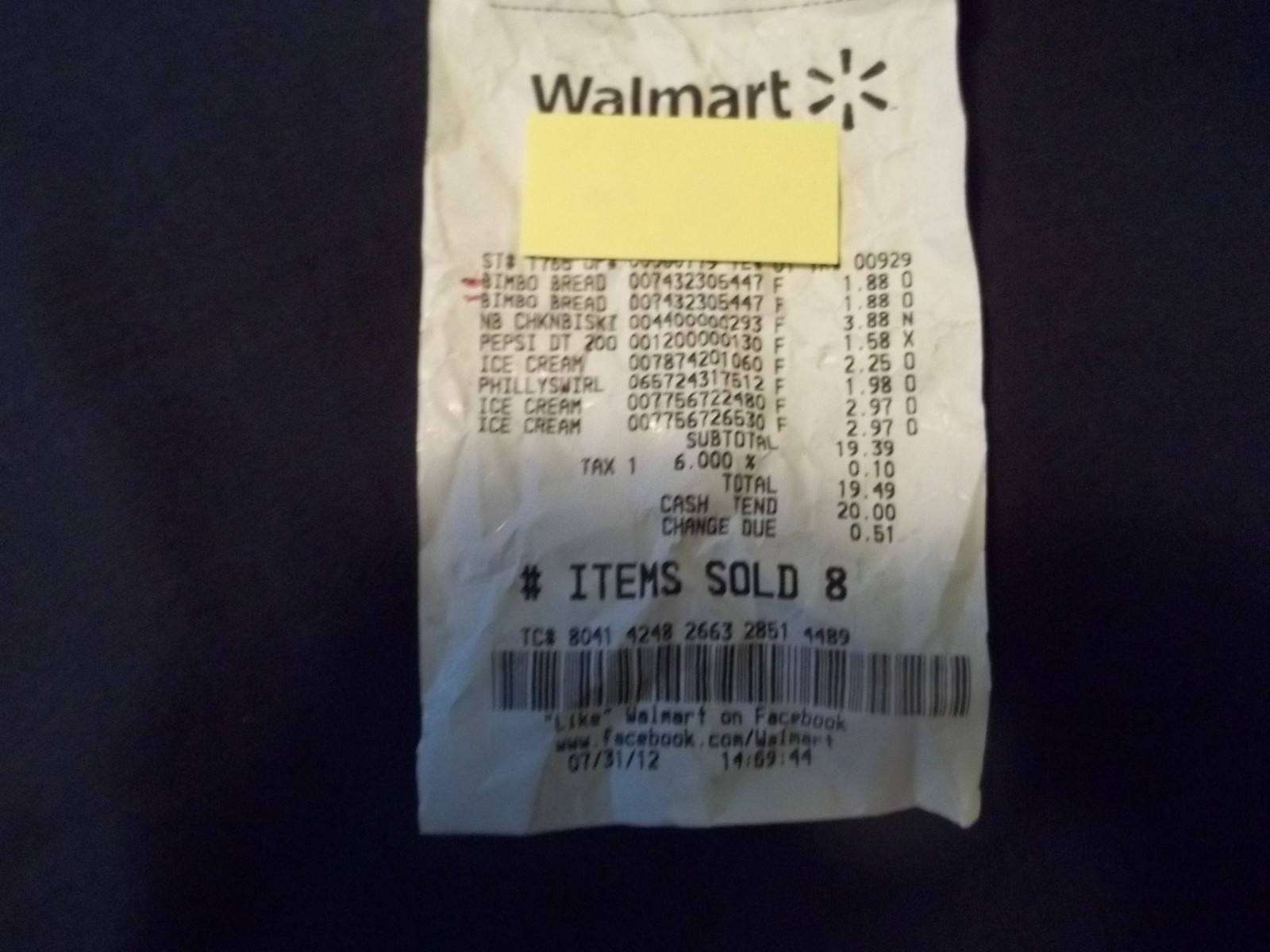The image features a white Walmart receipt centered against a black background, captured in close-up detail, making most of the information visible. A small, yellow Post-it note has been precisely cut to size and placed below the Walmart logo, obscuring some of the store's address and other identifying details. Next, the receipt lists the items purchased, with two specific entries—Bimbo bread—highlighted by a small red pen mark on the left side, possibly indicative of someone's tracking effort. Each Bimbo bread costs $1.88. The receipt shows a total of eight items purchased on July 31st, 2012. Among the items bought are three ice creams, one Pepsi, a Philly Swirl, a cheesecake, and a chicken sandwich, suggesting a shopping trip focused on a mix of frozen treats and comfort food.